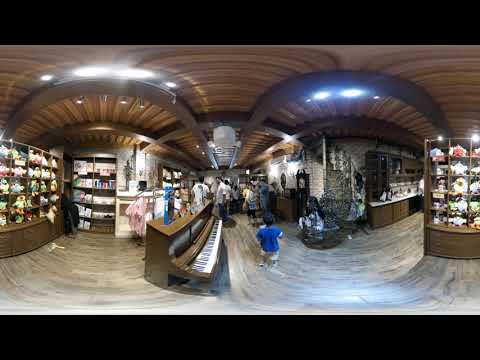This image is a distorted panoramic view of the interior of a store, seen through two fisheye lenses, one on the left and one on the right. The store features wooden cabinets and shelves lined with various objects, including figurines and stuffed animals. Alongside these, there are more shelves that appear to hold books. In the center of the frame, an upright piano with additional items on top stands prominently. To the right of the piano, a little boy with dark hair is wearing a blue shirt and beige or yellow shorts, while a little girl sits on a stool or table to his right. The adults in the background are either shopping or preparing to check out. The wooden ceiling and mottled brown and beige floor add to the indoor ambiance of the scene. Ceiling lights and shelves filled with items hint at a bustling, organized environment filled with varied colors such as white, royal blue, black, green, yellow, red, brown, dark brown, and tan.